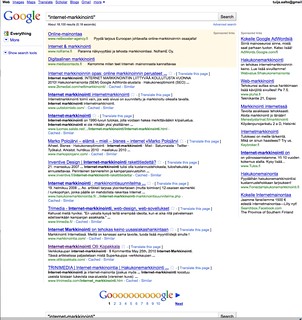A screenshot of a Google search results page. The iconic multicolored Google logo—blue "G," red "O," yellow "O," blue "G," green "L," and red "E"—is positioned at the top left corner. Below the logo are navigation options labeled "All" and "More." The search results page comprises ten links, although the text is illegibly small. The first three links are highlighted in a pink box, likely indicating they are sponsored ads. At the bottom of the page, there's an elongated "Goooooooooogle" text accompanied by a forward arrow, providing pagination options numbered 1 through 10. Additionally, a "Next" button is available for navigating further search results. Attempts to zoom in blur the text, making it challenging to discern the search query or link details.